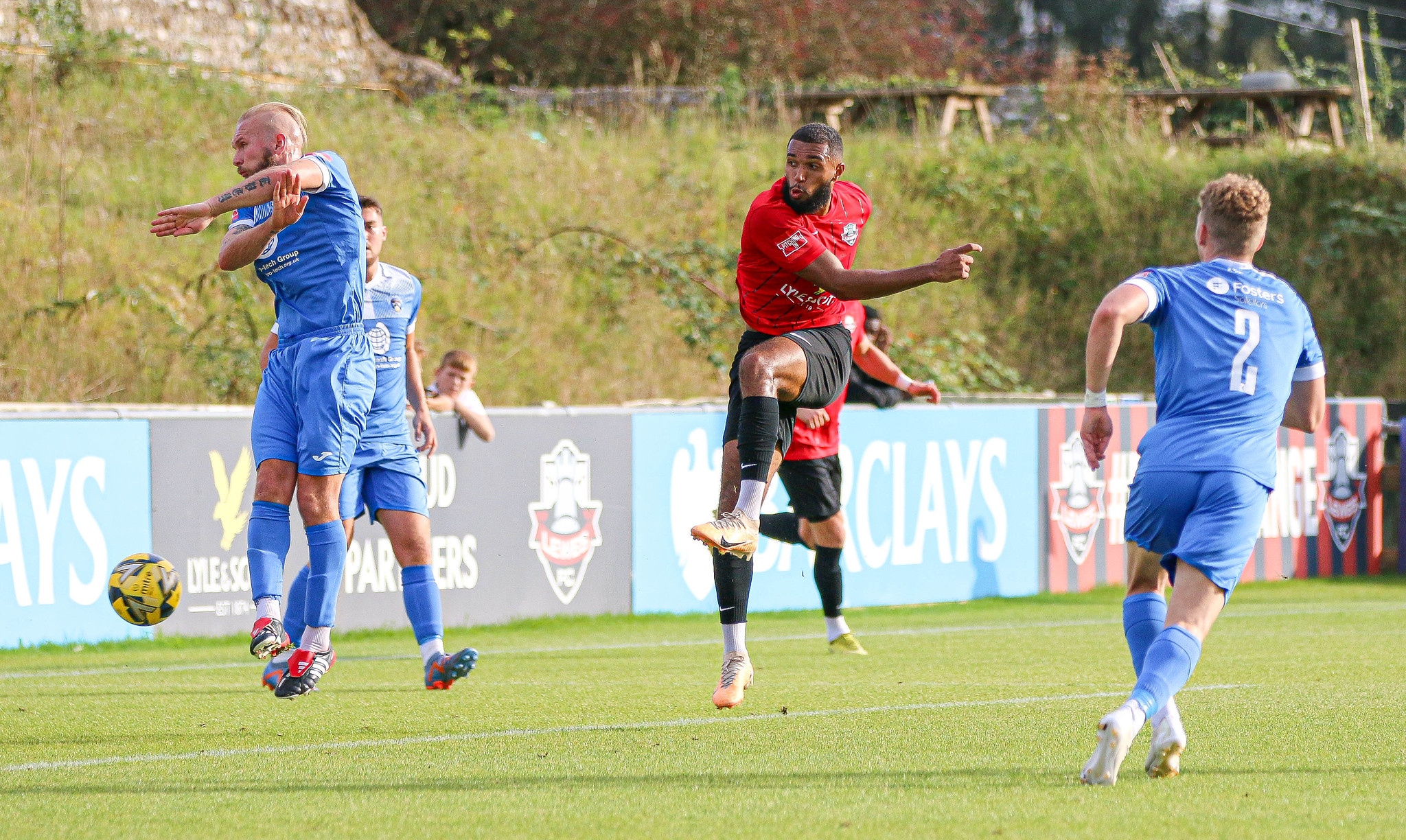This is a vivid, full-color photograph capturing an outdoor soccer match on a sunny day. In the image, five players are actively engaged on the pitch. Three of the players are donning bright powder blue kits, which include matching blue jerseys, shorts, and socks, with their boots being a combination of red and black. The other two players are from the opposing team, distinguishable by their striking red and white kits. One key player in the center is outfitted in a red jersey, black shorts, black socks, and white boots, notably sporting a visible white Nike Swoosh on his shin guard or sock. The soccer ball being contested is uniquely black and yellow, adding contrast to the scene.

The surrounding environment features various advertisements along the side of the pitch. The most prominent is a blue Barclays sign with white lettering, while another ad, obscured partially behind a player, is striped orange and blue. Beyond these advertisements, a grassy hill ascends, capped with a wooden table at its crest. A young boy can be seen watching the match intently from behind the advertisement wall, adding a touch of local community involvement to this dynamic scene.